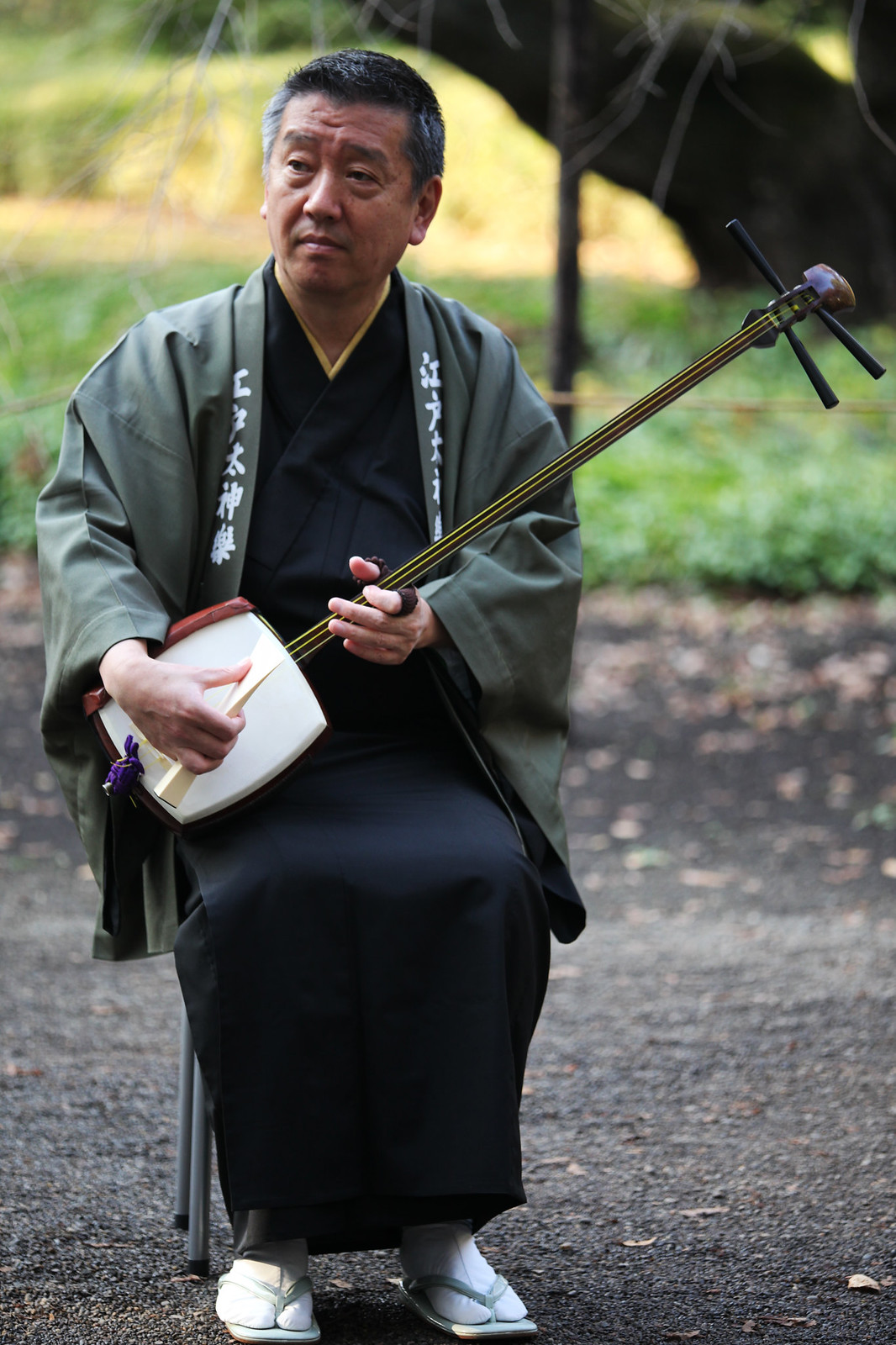The photograph depicts a middle-aged Asian man seated in a black-capped, gray metal chair on a paved or tarmac surface. Behind him, a large green field with towering trees stretches out, creating a serene outdoor setting. The man has black hair flecked with grey and wears a distinctive green coat adorned with Asian characters along the lapels. His attire also includes a long black robe extending from his neck to his ankles, and he sports white socks with orange thong sandals on his feet. In his hands, he holds a shamisen, a traditional Japanese three-stringed instrument with a long, slender neck and a white, semi-square body edged with red wood, played using a large pick.